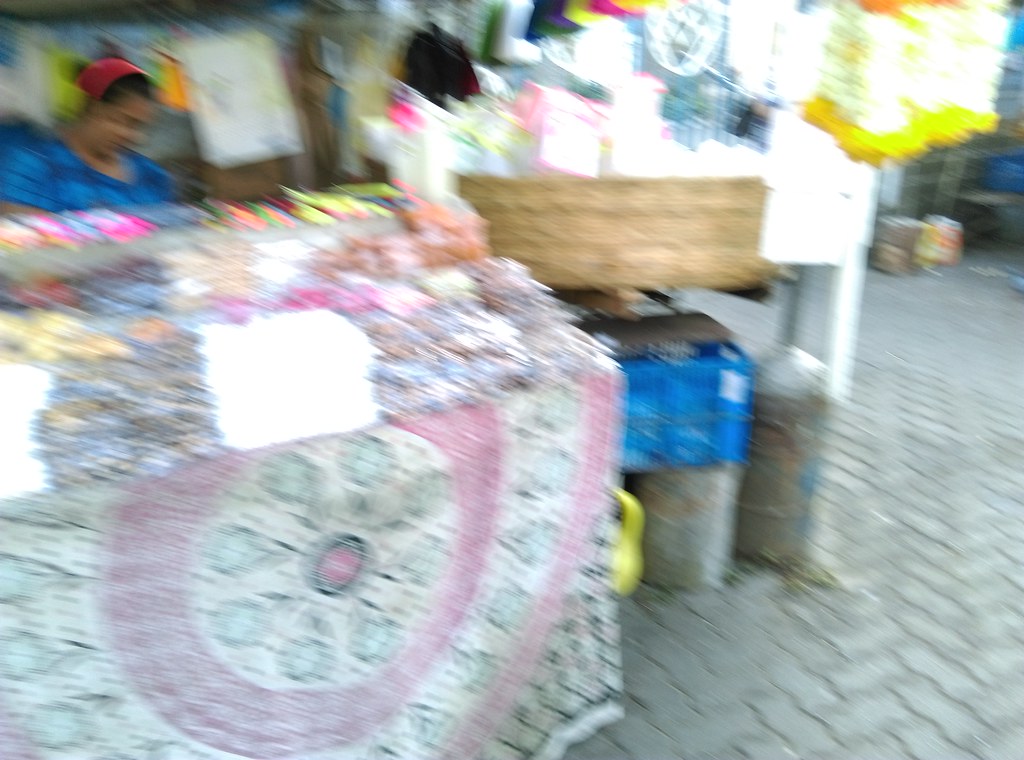This image, though blurred with motion, captures the vibrant scene of a traditional market stall, possibly located in a picturesque South American town. The full-color photo reveals a cobblestone-tiled ground setting the stage for the lively atmosphere. On the left side of the frame stands a market stall adorned with an intricately patterned, ornate fabric cloth draped over the front of the table. Despite the motion blur that obscures the details on top of the table, the indistinct shapes and blobs suggest an assortment of food items, possibly pastries or other local delicacies. Behind the table, a woman dressed in a vivid blue blouse and adorned with a striking red head wrap tends to the stall, adding a touch of human warmth to the bustling market environment.